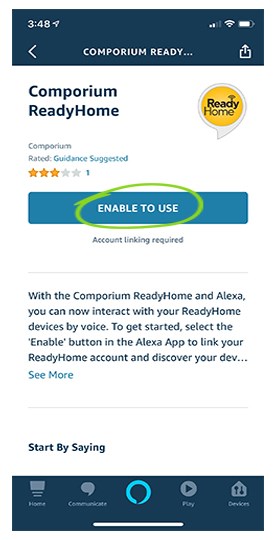The image depicts a cell phone screen with a navy blue header at the top. On the top left side of the header, the time is displayed as "3:48," accompanied by a location icon. To the right of the time, there are two bars indicating internet connectivity, three bars for Wi-Fi signal strength, and a fully white battery icon. An arrow pointing to the left is also visible in the header. 

In the middle of the header, the text "Comporium Ready" is displayed, alongside a share icon. Below the header, a section with a white background and blue text reads "Comporium Ready Home.” To the right of this text, there is a "Ready Home" logo—a white speech bubble with a yellow circle in the middle and the words "Ready Home" inside it.

The text below the logo reads "Comporium Rated: Guided Suggested," followed by three stars. A blue button labeled "Enable" with a green circle around it is prominently displayed. Below this button, text reads, "With the Comporium Ready Home and Alexa, you can now interact with our Ready Home devices by voice. To get started, select the enable button in the Alexa app to link your Ready Home account and discover your IDEV and see more."

After another dividing line, the text continues, "Start by saying," but the example phrases are cut off by a dark navy bar at the bottom of the image. The navigation bar at the bottom of the screen includes icons labeled "Home," "Community," and "Communicate," with a light blue circle in the center. Other icons include "Play" and "Devices."